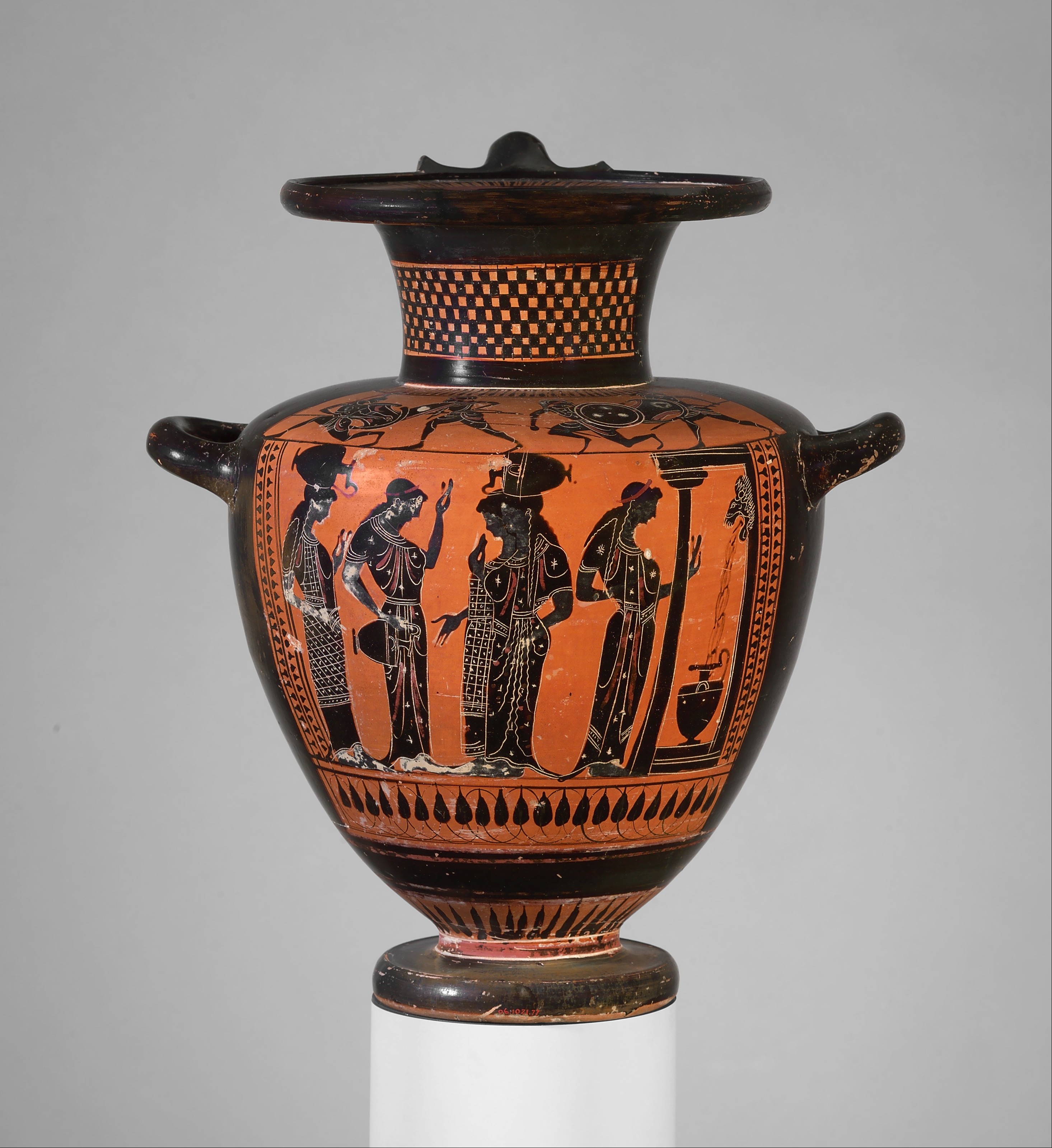The image displays a predominantly black vase featuring intricate orange designs, likely photographed in a museum or as a product listing. The vase is adorned with detailed depictions of ancient Egyptian figures, highlighting a vivid scene. On one side, four women are illustrated, each engaged in carrying vases, with one balancing a vase on her head, another holding one in her hand, and a third gathering water under a spout. Above these women, black figures of men with shields and spears are depicted amidst battle on an orange background. Additionally, another side portrays four Egyptian figures near a frame or doorway. One man dons an unusual headpiece and another holds a scepter behind his back. A deity, possibly Osiris, stands with a staff, and another individual holds fire. The vase is positioned on a white stand, complemented by a small black handle on its side, enhancing its antiquated and ornate appearance. This detailed scene encapsulates themes of daily life and mythology in ancient Egypt.